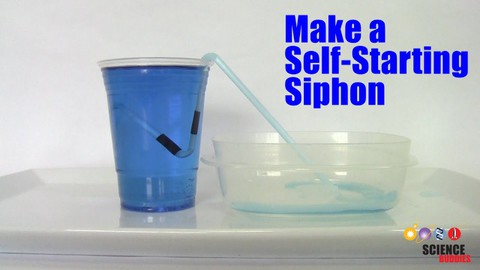The image depicts a detailed science project for constructing a self-starting siphon. The title "Make a Self-Starting Siphon" is prominently displayed in bright blue text with a white border at the upper right corner. The setup includes a clear plastic cup filled almost to the brim with blue liquid. A straw, featuring black sections, is submerged in the liquid, bending into a V-shape and rising again to exit the cup. The end of the straw then extends downwards into a plastic Tupperware container, which appears to hold some of the transferred blue liquid. All items are placed on a white ceramic tray. The bottom of the image displays a colorful logo for "Science Buddies," incorporating various hues like yellow, purple, blue, and red.